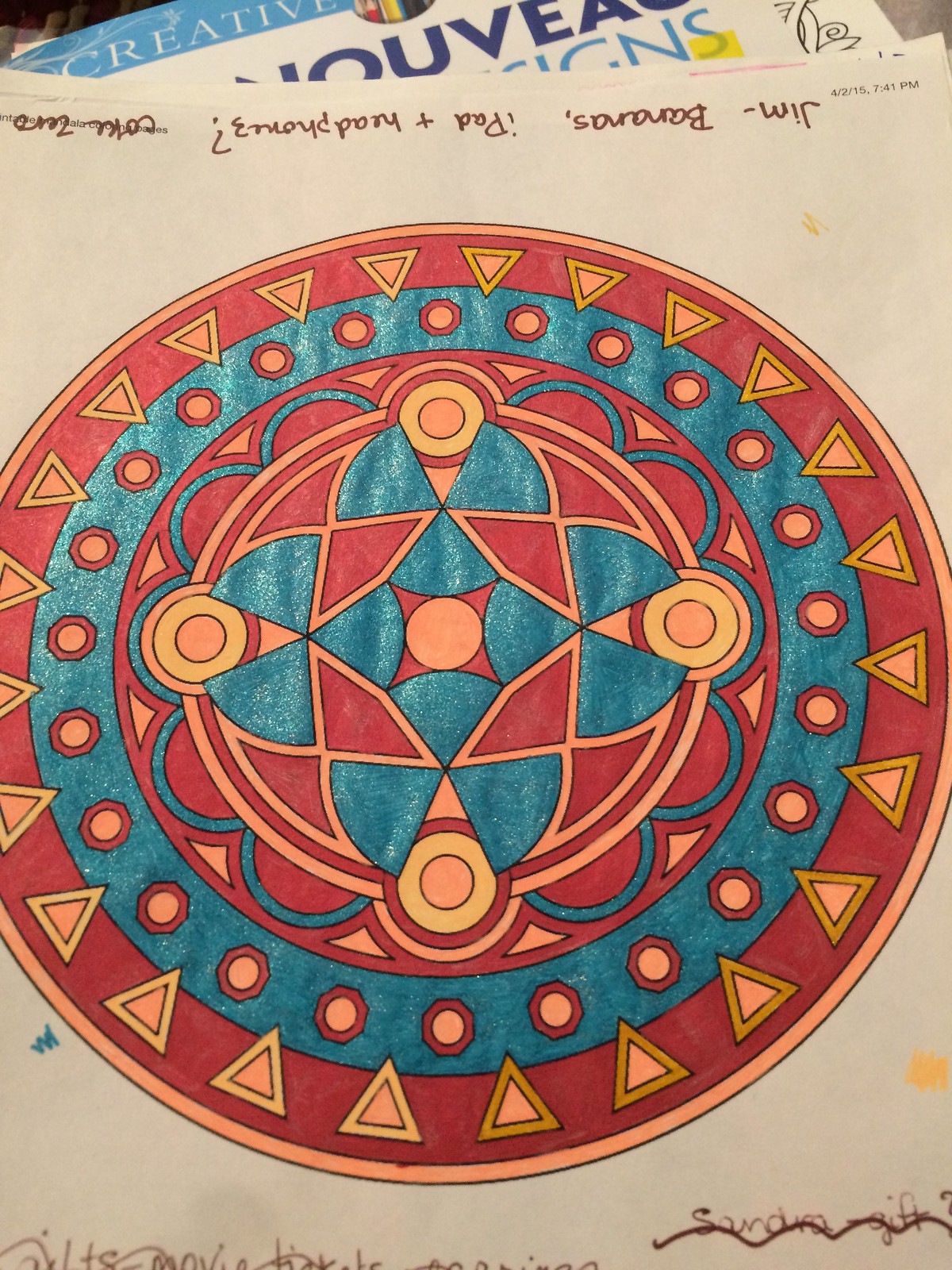A vibrant and meticulously designed worksheet, likely originating from an art or creative class, is depicted. At the top of the page, handwritten or typed text reads "Jim Barnabas iPad + headphones?" along with "Coke Zero." The central focus of the worksheet is an intricate geometric design prominently featuring a round shape adorned with a variety of smaller geometric elements, including triangles, circles, and half-circles. The design is vividly colored with an impressive array of hues: striking red, warm yellow, radiant orange, and a strikingly unique metallic blue. The precision with which the design is executed suggests either a high level of skill or a printed origin, and it evokes a distinct aesthetic reminiscent of traditional Indian geometric patterns.